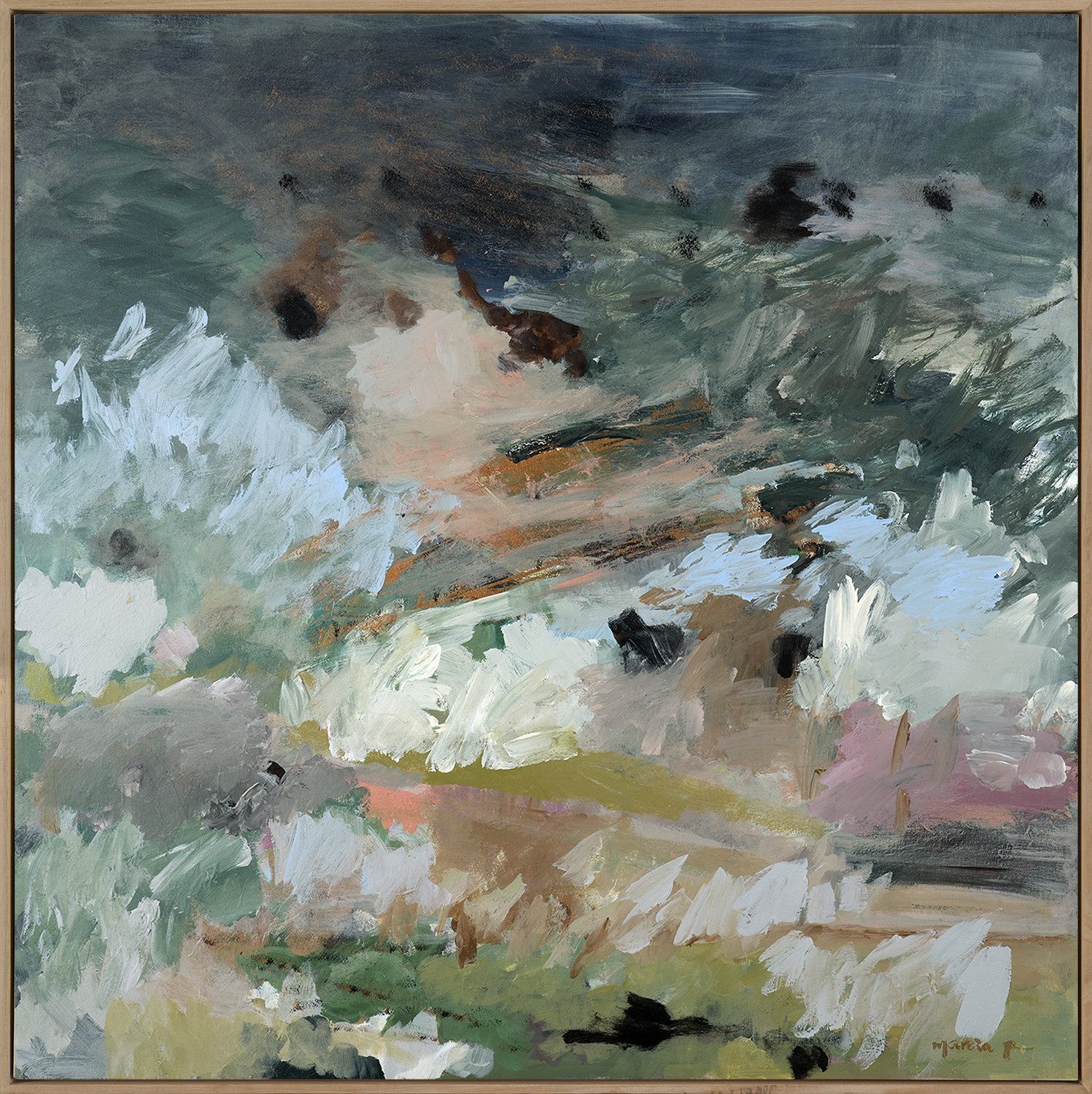This image showcases an abstract oil painting on canvas, encased in a light tan gray frame accented with a black line. Predominantly composed of a turquoise or dull turquoise gray-blue, the artwork features a harmonious blend of colors, including dark green, white, light blue, lime green, olive green, forest green, brown, beige or cream, and peach, with hints of pink and black. The composition employs dynamic brush strokes and splashes, evoking the sense of waves breaking against rocks, though it remains largely non-representational. The painting's square shape further enhances its balanced yet spontaneous aesthetic, highlighted by brushes of color that sweep across the canvas in various shapes and angles, creating a vibrant, natural, and earthy palette.